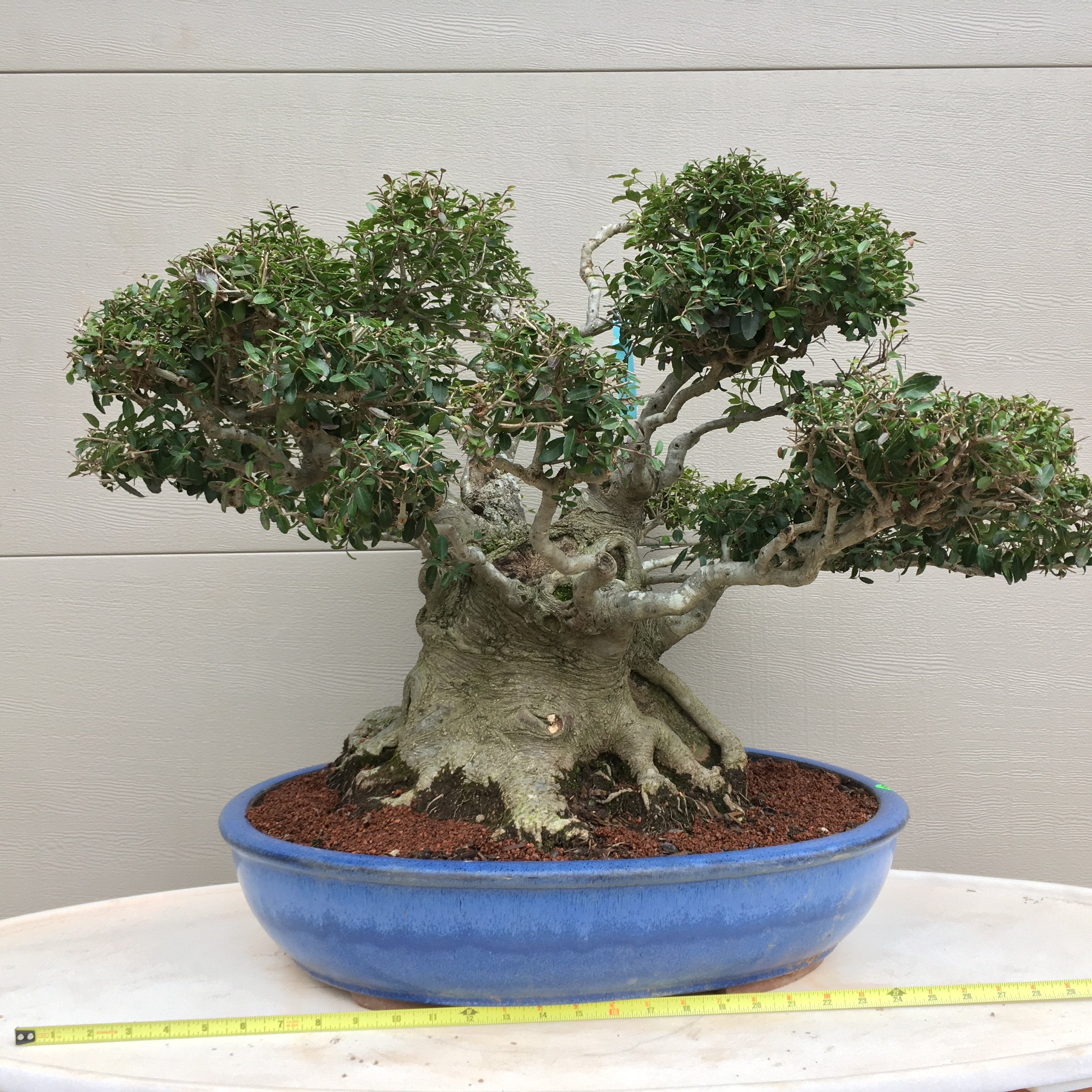A vibrant, square, outdoor photograph captures a striking bonsai tree displayed on a round, white stone table. This meticulously groomed tree features a thick, gnarled brownish-gray trunk with thin branches that fan out, adorned with vivid green leaves. Root tendrils intricately spread across the topsoil, housed in a large, blue ceramic pot filled with rich, brown dirt. The cool pot rests centrally on the table, beneath which a yellow measuring tape stretches horizontally across the image's bottom, indicating the pot's diameter is approximately two and a half feet. The serene backdrop is a painted, light gray wall featuring wide, horizontal wooden planks, contrasting softly against the bonsai’s natural elegance.